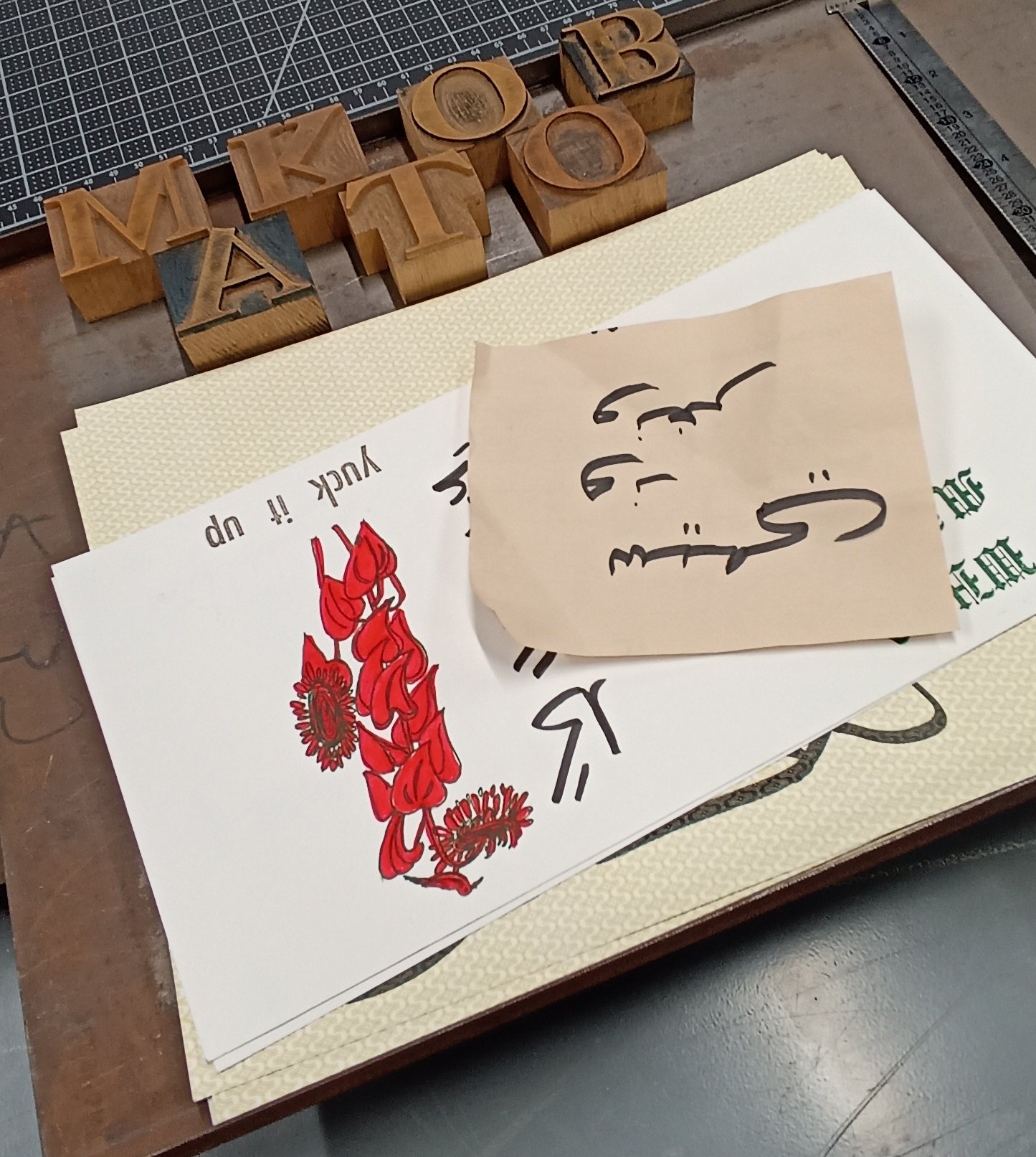In this detailed image, we are looking down at a creative work table arranged with various tools and materials. Dominating the scene is a black board featuring grid patterns, white lines, and built-in measurements such as a ruler or yardstick. To the right of the board lies a silver metal ruler, accentuating the workspace's precision. On this brown wooden table, which rests on a gray concrete-like surface, are five wooden stamps used for printing, displaying the letters M-K-O-B-A-T-O with some bearing smudges of black ink suggestive of recent use.

Amidst these tools, a series of stacked papers catch the eye. At the top, a tan paper inscribed with what might be Farsi or Arabic script partially covers the others. Below it lies a white paper adorned with a red flower design, and though the script beside the flower is partly obscured, the phrase "yuck it up" is legible. Additional layers include a yellowish-white paper with an indiscernible pattern. The overall scene vividly captures a moment in the creative process, blending traditional printing tools with multicultural written expressions.